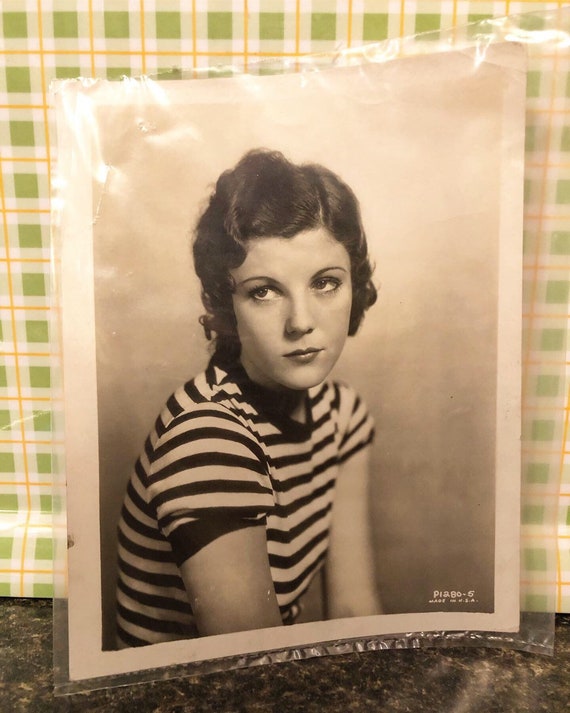This is a detailed photograph of an old black-and-white photograph that has been placed on a marble countertop adorned with a green, white, and orange checkerboard design. The original photograph, encased in a clear plastic protective sleeve, features a young woman with dark, slightly wavy, and short hair styled back, suggesting a possible era from the 1940s or 1950s. She is captured looking off to the side, seemingly with a neutral or slightly sullen expression, and her gaze is directed upwards to the right. Her well-groomed eyebrows add to the distinctiveness of her facial features. She is wearing a black-and-white striped t-shirt with dark cuffs and neckline, bearing a resemblance to a classic prison uniform or jersey top. The background of the photograph is a gradient gray that lightens towards the top, enhancing the strong shadowing in the image. The photo includes a small text inscription in the corner that reads "P1280-5, Made in USA". The overall appearance suggests it might be a vintage school photograph.